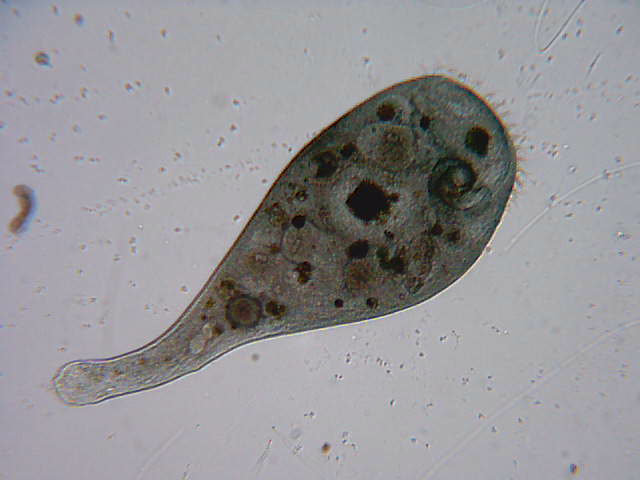This detailed microscopic image showcases a distinctively thick, teardrop-shaped, likely animal cell organism floating in a liquid medium. The background appears grayish, accentuating the organism which is viewed through a microscope. The organism's body is club-like with a prominent head and tapering tail. Its head features several small, thick hair-like projections or "fingers." Notably, a well-defined bullseye-shaped spot can be observed near the tail. The body of the organism appears somewhat transparent, revealing various internal structures or dots, possibly indicative of internal organelles or food particles. The image's overall color scheme is predominantly black and white, with subtle red tinting on one side, and a sharp clarity suggesting the use of high magnification. Additionally, tiny speckles and a small, worm-like figure are visible adjacent to the main organism, enhancing the image's intricate detail.